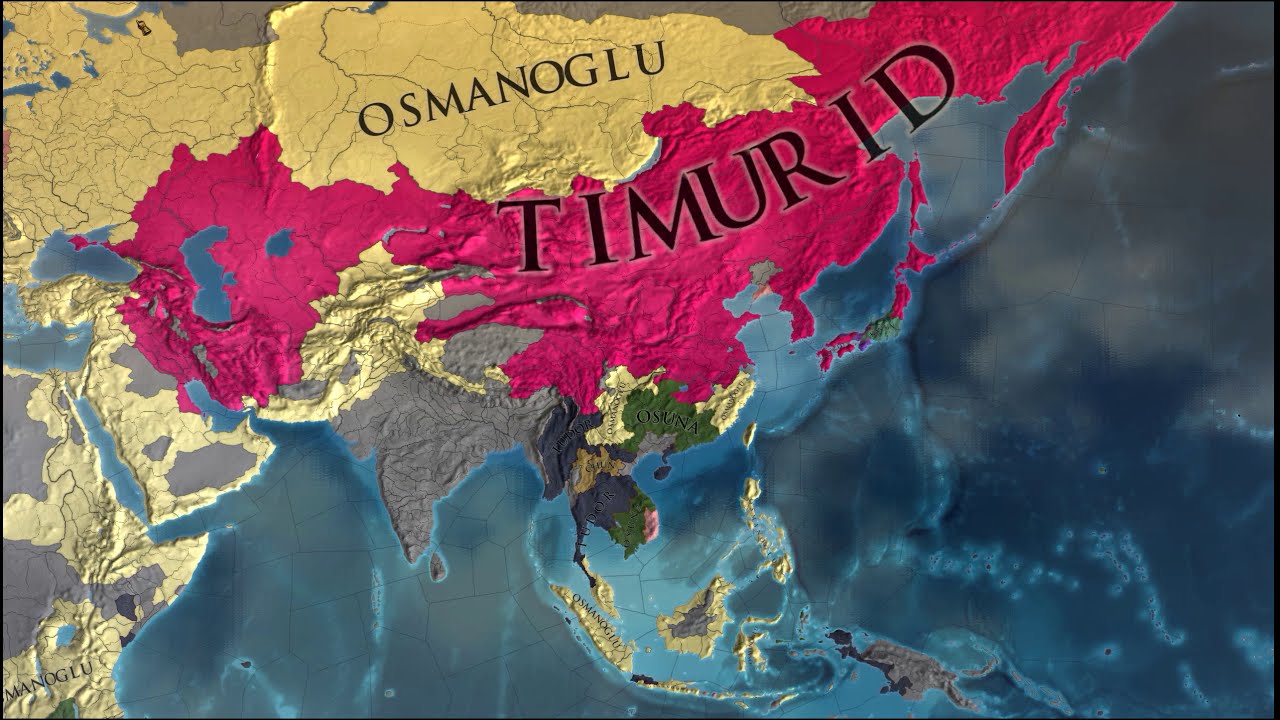The image depicts a detailed and textured 3D map focusing on extensive regions including Asia, the South Pacific, the Middle East, the eastern part of Europe, and the northeastern part of Africa. The landmasses are vibrantly colored to signify different areas of control or interest, with hues of yellow, red, green, dark blue, gray, and even purple. The ocean surrounding these territories is shaded in various blues, enhancing the map’s depth. Prominent regions are labeled with unique names; the sizeable golden area in the top middle is marked "Osmanoglu," and a striking red region is labeled "Timurid." Another key area is marked with "Timur," possibly corresponding to what modern maps identify as Asian Russia. The map appears to embody an alternate cartographic representation, potentially from a game, overlaying Earth’s geographic features with distinct nomenclature and territorial boundaries.